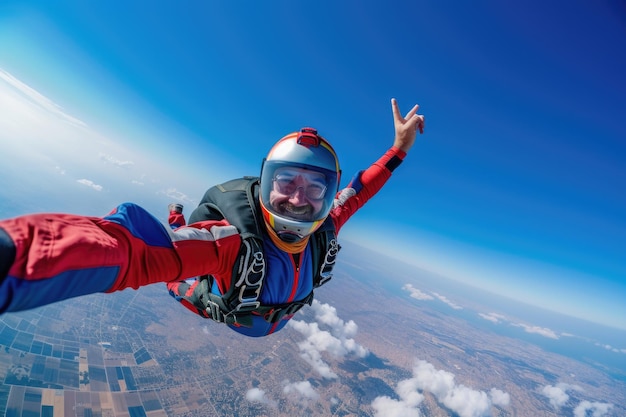In this dynamic and exhilarating close-up photograph, a skydiver is captured mid-fall, taking a selfie with his left arm outstretched, holding the camera at the end. He is clad in a striking red skydiving jumpsuit accented with blue patches and a distinctive white stripe. His black parachute pack, not yet deployed, is strapped securely to his back. On his head, he sports a clear-visored helmet with gray sections and vibrant red and orange stripes, under which he appears to be wearing glasses, and his beaming smile is clearly visible.

His right hand is raised, forming a peace sign with extended fingers, adding a playful element to the intense moment. The sky behind him is a deep, dark blue, seamlessly transitioning into misty fog and cloud cover below. Puffy white clouds surround him, with some floating to his right in an enchanting cyan sky. Far below, the patchwork quilt of farmland displays a mosaic of beige, green, yellow, orange, and brown squares and rectangles, contrasted by smaller houses and a brown area to his far right. The horizon stretches out in the distance, enveloping this breathtaking skydive in the glow of daytime light.